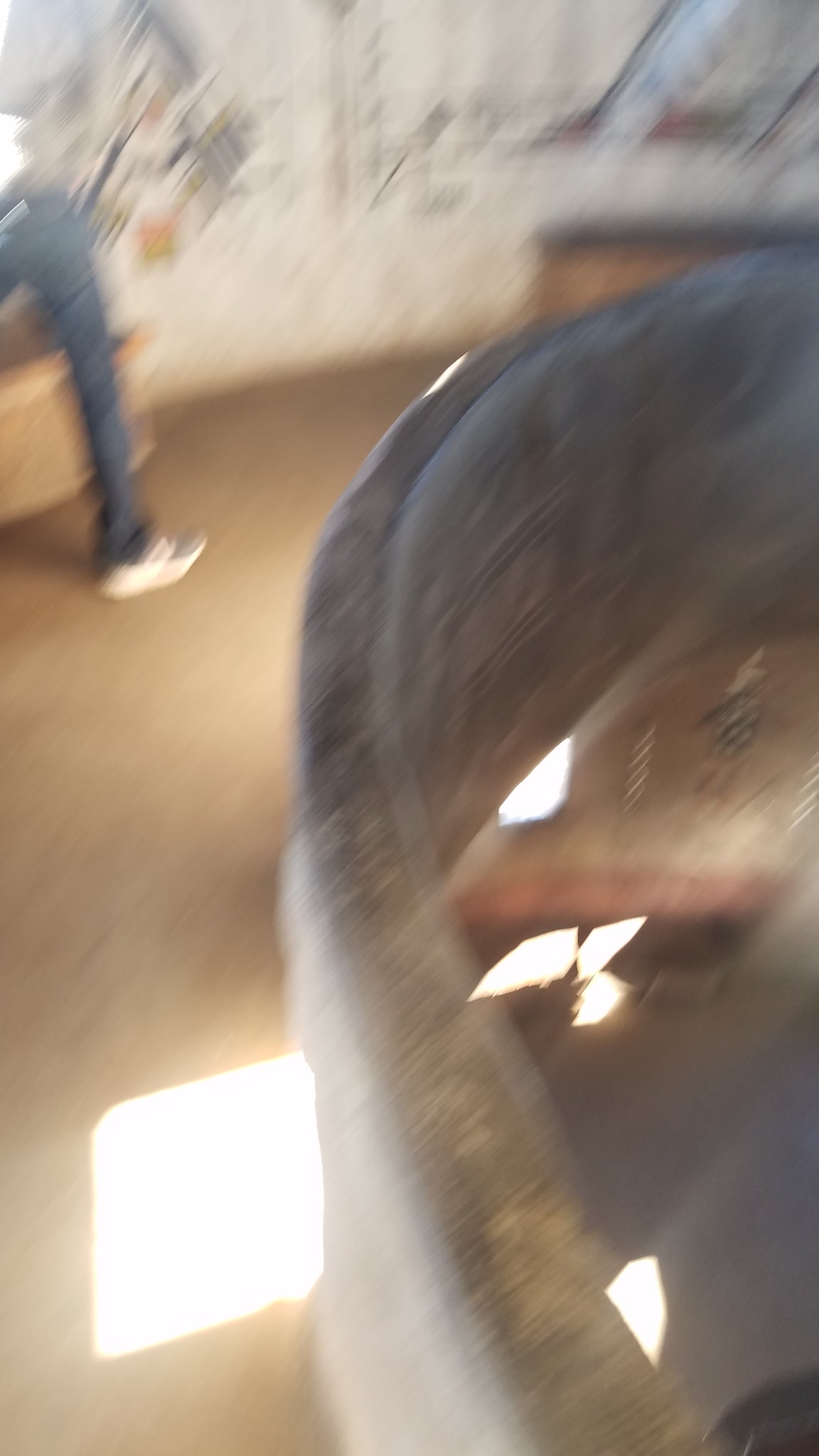The image captures an interior space with significant motion blur, creating a dynamic yet slightly disorienting effect. On the right side of the room, there is a large opening in the floor that provides a view of the floor below. A raised barrier encircles this opening, ensuring safety. The floor is covered in light brown carpeting, adding a subtle contrast to the scene. In the upper left corner, a person is partially visible, standing and gazing at something on the wall. They are dressed in blue jeans and a gray shirt, the latter almost blending into the off-white wall behind them, further obscured by the motion blur. The overall ambiance is one of movement and activity, despite the indistinct details caused by the blur.